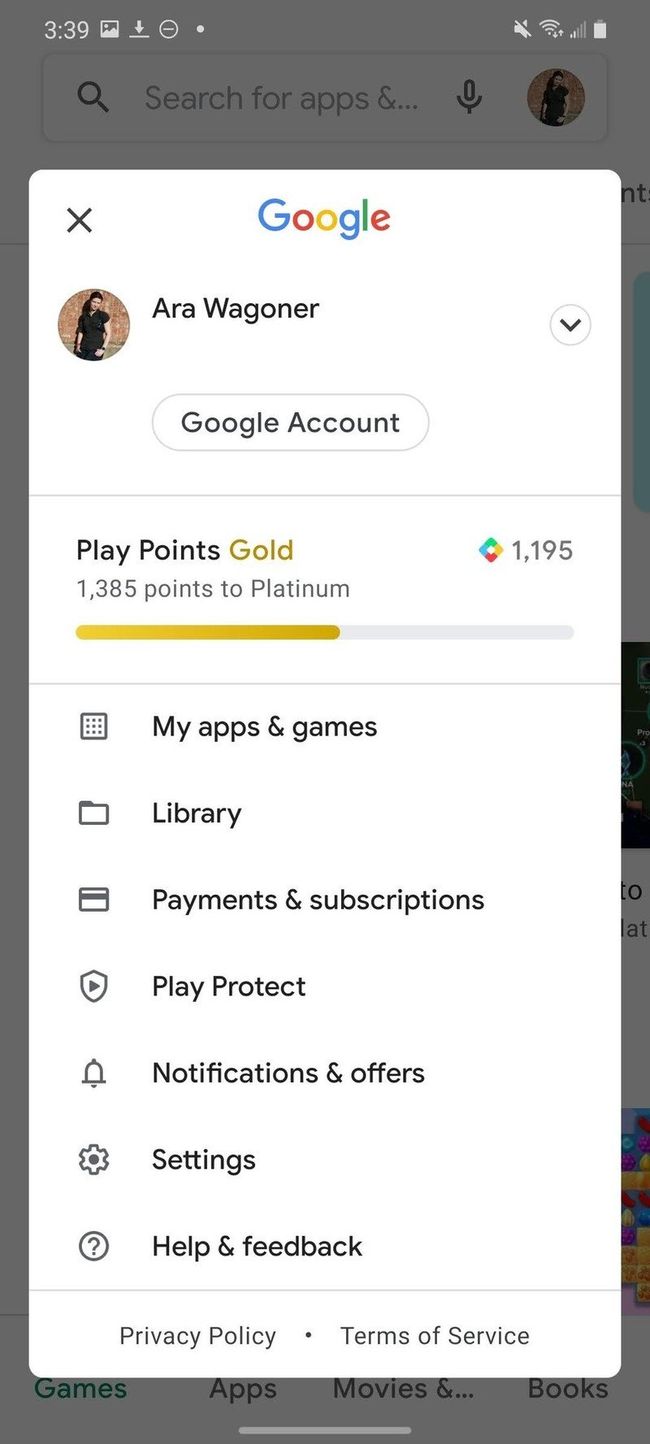This image captures an open Google account pop-up window overlaying a Google search page. The primary focus is on the pop-up window, which has a white background and a prominent gray-colored 'X' in the upper left corner for closing it. At the top center, the traditional Google logo is clearly visible.

Beneath the logo, a circular profile image of a woman with dark hair in a black shirt, standing against a brown wall, is displayed. Next to the profile picture, the name "Aria Wagner" is written in black font, with a phonetic spelling "A-R-A Wagner, W-A-G-O-N-E-R" just below it. The bold text "Google Account" is seen next, accompanied by a clickable button.

Further down, the user’s Play Points balance is displayed as "Gold 1195" with "1385 points to platinum." A list of selectable options follows, including "My apps and games," "Library," "Payment and subscription," "Play Protect," "Notifications and offers," "Settings," "Help and feedback," "Privacy policy," and "Terms of service."

In the gray background portion, the upper section includes a search bar. The status bar at the top of the screen shows the current time (3:39), battery level, and indicators for data and Wi-Fi connectivity located in the upper right corner.